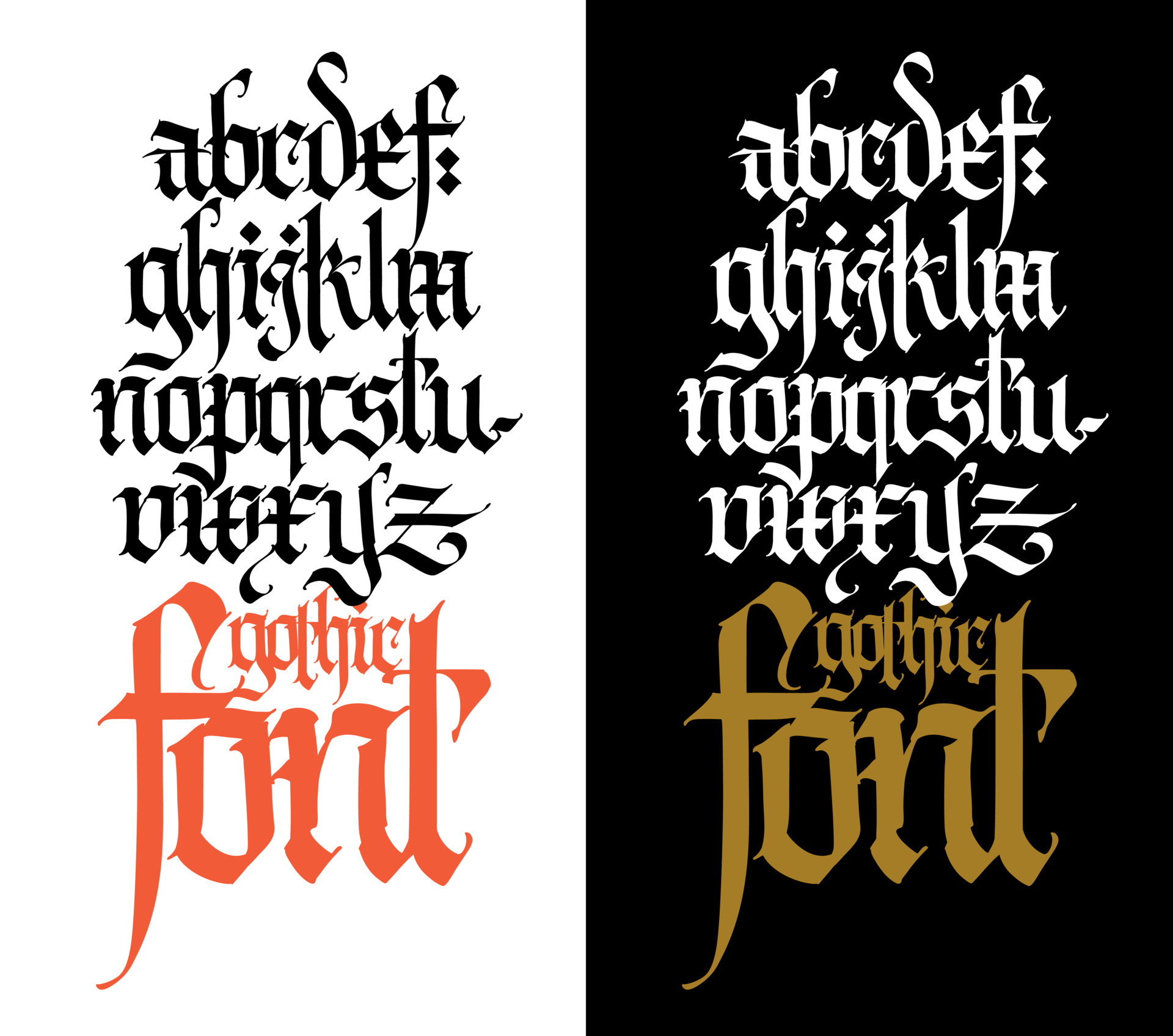The image displays an alphabet chart in two color schemes. On the left, a white background features black text that presents the letters A to Z arranged in rows. The first row has A to F, the second row G to M, the third row N to U, and the fourth row V to Z. Below the alphabet, the word "Gothic" appears in small red text, followed by a much larger word "Font" in the same color. On the right, the same alphabet is shown, but with a black background and white text. At the very bottom, the word "Gothic" is written in dull gold, slightly smaller than the alphabet letters, while the word "Font" is again much larger, approximately twice the size of the other text elements.